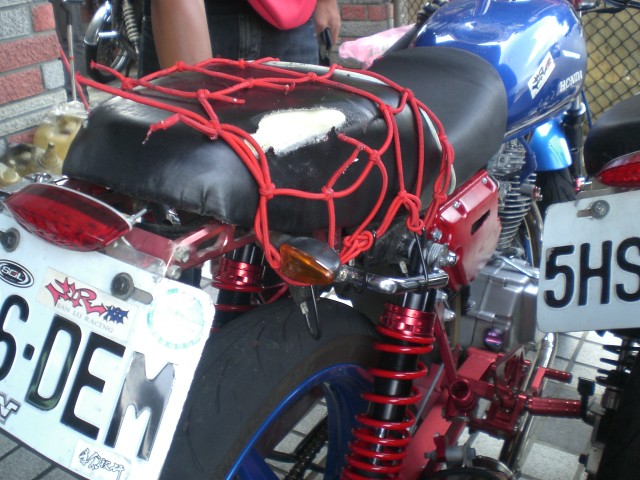This photograph captures a detailed rear view of a blue Honda motorcycle, prominently showcasing various elements. The motorcycle's black seat is divided into a main rider's section and a shiny-backed passenger seat adorned with red netting. The bike also features red coiled shocks and fairly thick, black tires with blue rims. Two license plates are visible: one at the rear reading S-R S-D-E-M, and another on the right side saying 5-H-S. The front part of the motorcycle, which also has blue accents, displays some white text, likely the brand name Honda, though part of it is obscured. The background reveals a mixed urban setting with a red and white brick wall, a chain-link fence, a yellow object resembling a tank, and gray tile pavement. There is a person, partially visible, wearing dark shorts and holding a phone, standing next to the motorcycle. The photograph appears to cut off some parts of the image, not fully displaying the handlebars nor the entire license plates. A similar motorcycle is partially visible on the right side of the image, and there is a red reflector light and additional red details present.